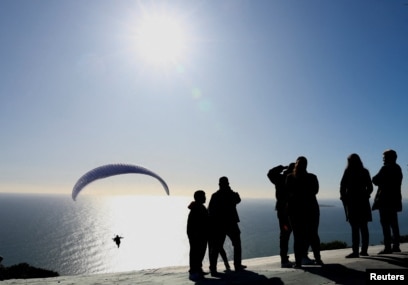A Reuters photograph, taken outdoors, captures a serene yet striking moment as a paraglider, with a blue parachute, glides low over a vast expanse of shimmering sea. The bright morning sun, positioned in the sky at the center left, casts a dazzling reflection on the water. Silhouetted against the light, about six onlookers stand in profile on a gray hillside, their forms rendered almost completely black by the sun's intense glare. In the distance, a small island barely peeks out from the horizon, which is tinged a faint yellow, suggesting the early hours of the day. The clear blue sky enhances the tranquility of the scene, while a Reuters watermark sits unobtrusively in the bottom right corner.